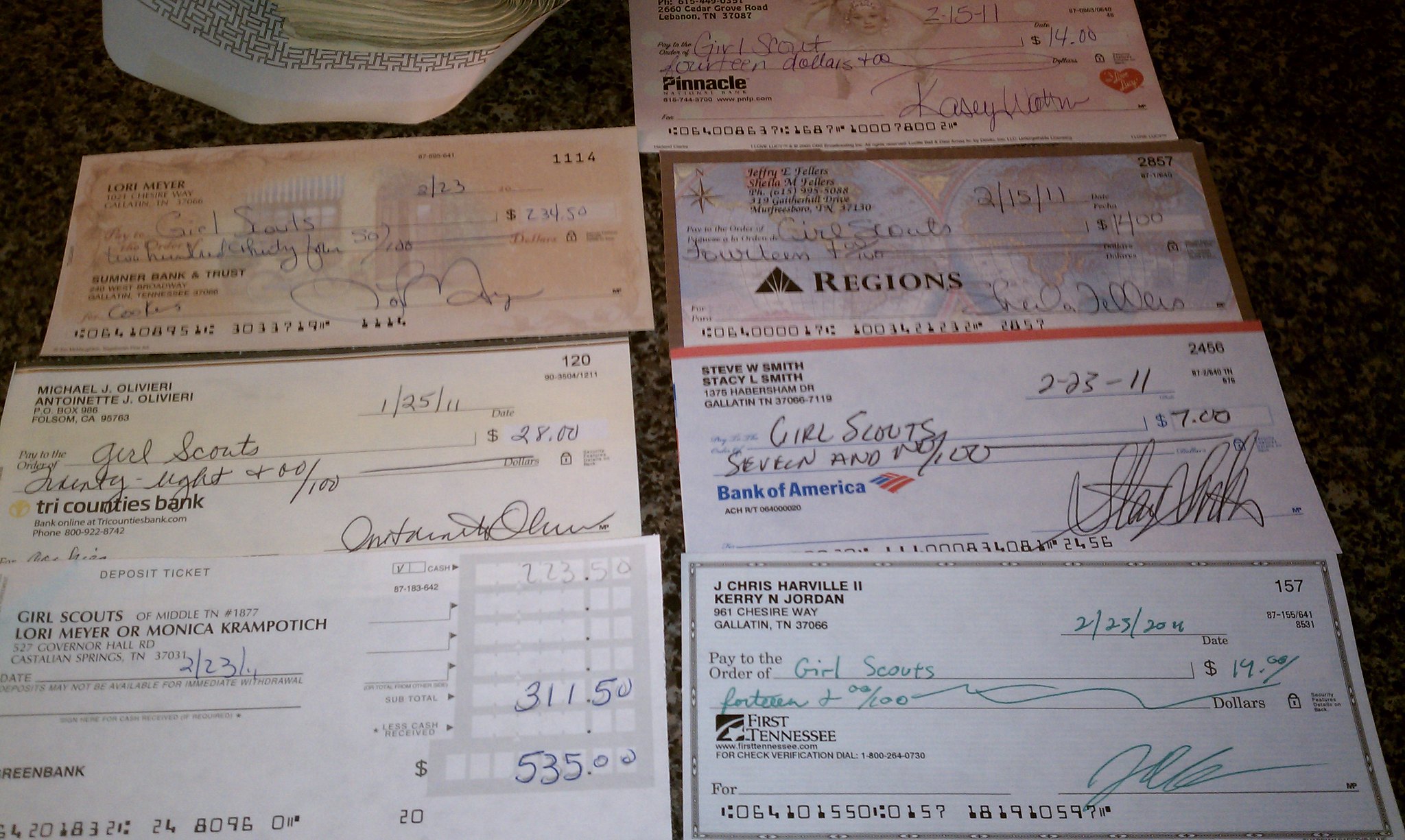This color photograph captures a countertop in a dark brown shade with subtle beige specks, prominently displaying a cluster of personal checks and an envelope. The black and brown countertop holds an envelope, slightly ajar, revealing crumpled bills inside. Surrounding the envelope on all sides are seven different checks, all made out to the Girl Scouts, reflecting contributions from various donors. The checks feature a spectrum of colors and designs: an orange check with indistinct characters, a yellowish check, a pink check with a heart emblem, a blue check with a red border, a white check from Bank of America, a green-tinted check from First Tennessee, and another from Regions Bank. Each check is directed towards the same cause, likely for Girl Scout cookies, with amounts varying—$19, $7, $28, $14, and another for $14. Additionally, there is a deposit slip at the bottom left corner labeled 'Girl Scouts of America,' indicating a total deposit sum of $535.